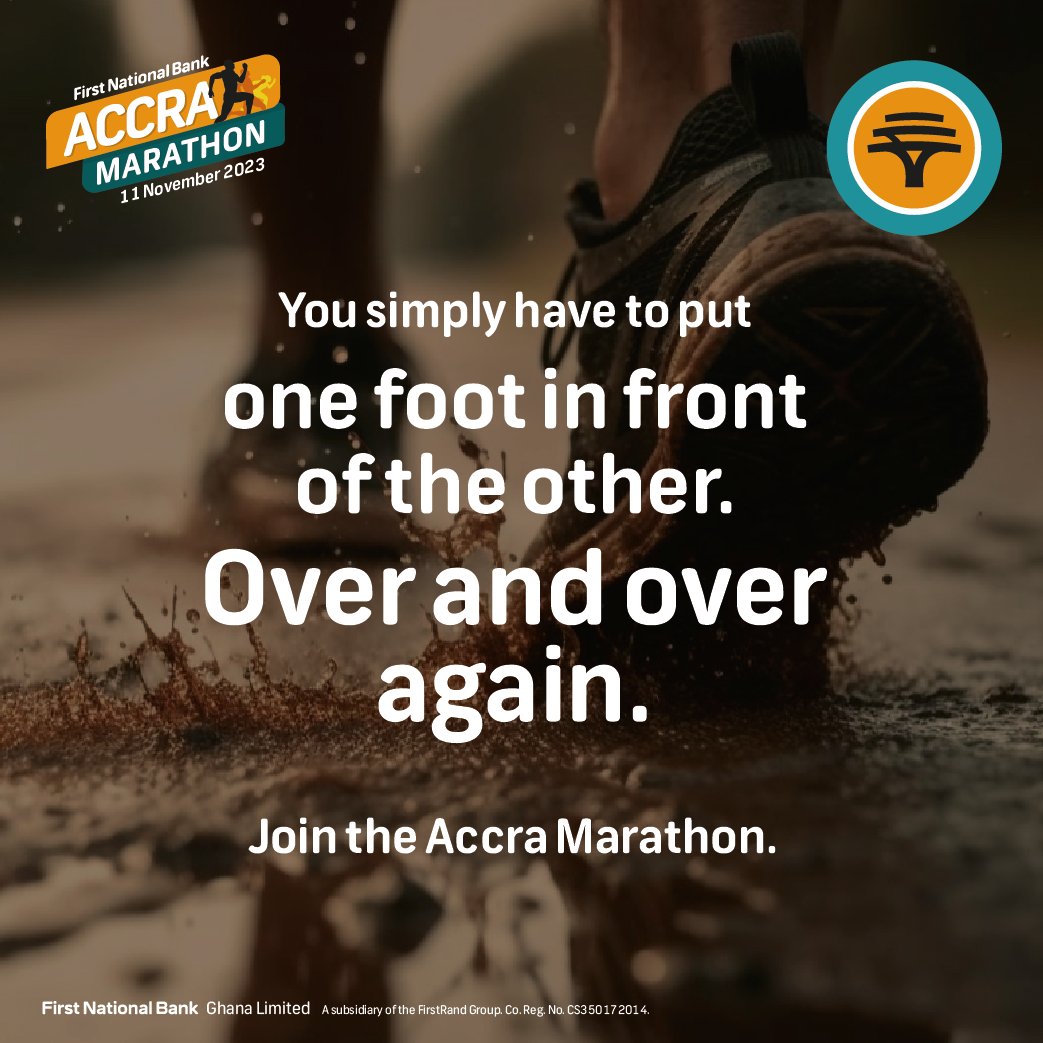The image is a square-shaped poster primarily in shades of brown and beige, suggesting a rainy or muddy setting. At the center, two feet in light blue shoes are mid-stride, walking through a puddle, with reflections of distant trees visible in the water. Superimposed in the center in white text is the motivational phrase: "You simply have to put one foot in front of the other over and over again," followed by "Join the Acro Marathon." The upper left corner features the First National Bank logo alongside yellow and blue rectangles that detail the event: "Acro Marathon, 11 November 2023." The upper right corner holds a circular emblem bordered in blue, showcasing a black tree. In the lower left corner, additional text indicates First National Bank's sponsorship and legal registration details. The overall feel is one of determination and endurance, encapsulated by the muddy, wet environment.